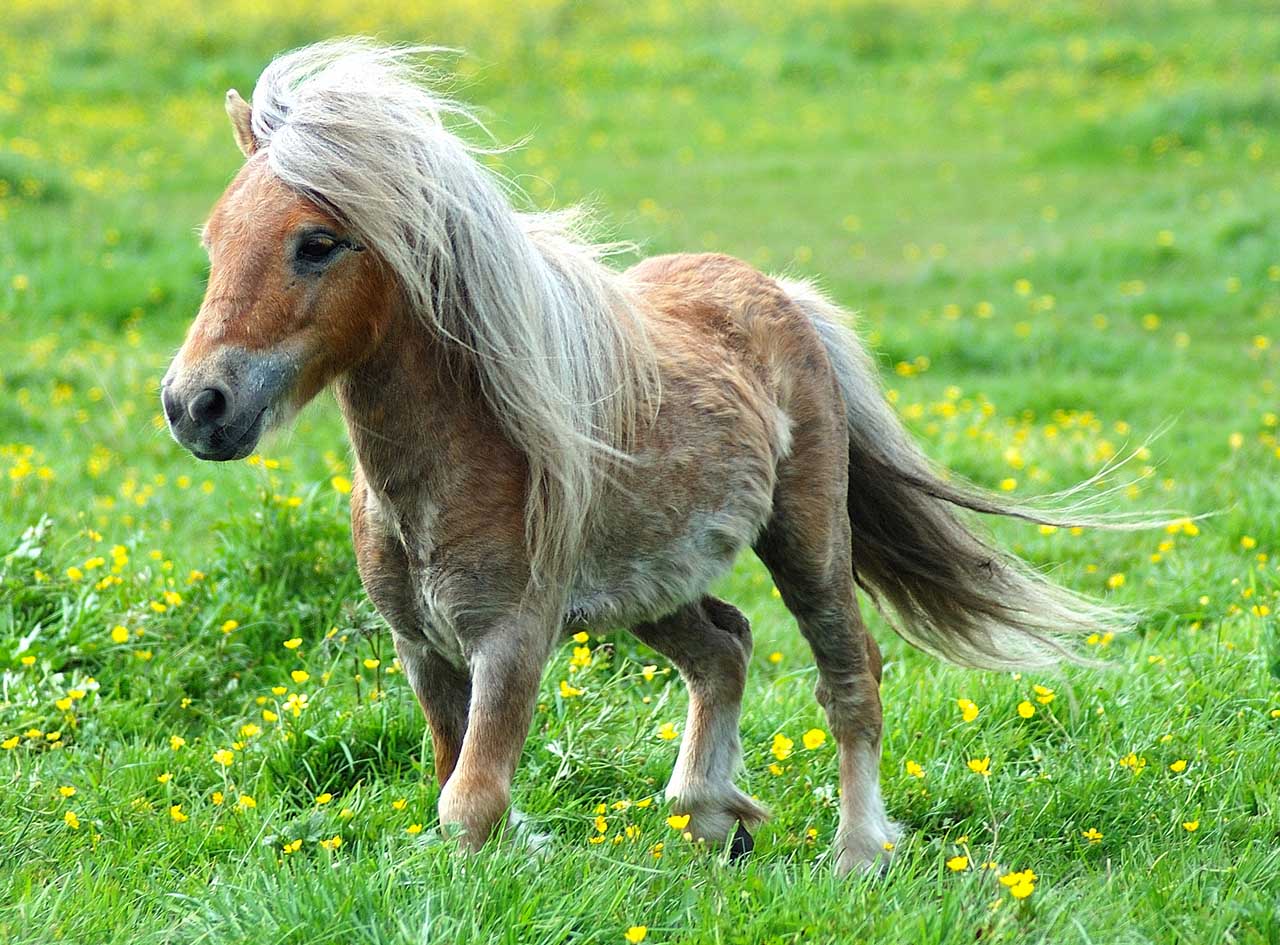A bright green field scattered with little yellow wildflowers sets the stage for a charming scene featuring a content and spirited miniature horse. The horse, an orangish-brown dwarf breed, appears to be trotting or running to the left, showcasing its playful nature. Its mane, a mix of long tan and grayish-white strands, cascades over the left side of its face, partially obscuring one short ear. The horse's head is predominantly medium brown with noticeable graying around the nose and eyes, adding character to its expressive face. Its body continues the orangish-brown hue on top, transitioning to white on its underside and legs. The legs are mostly brown except for the ankles, which are white, matching the white patches on its belly and neck. Its tail mirrors this coloration, blending brown and grayish-white. The image, with a slightly blurry background, captures the lively essence of this miniature horse amidst the lush ankle-high grass and scattered wildflowers, exuding a feeling of joy and freedom.